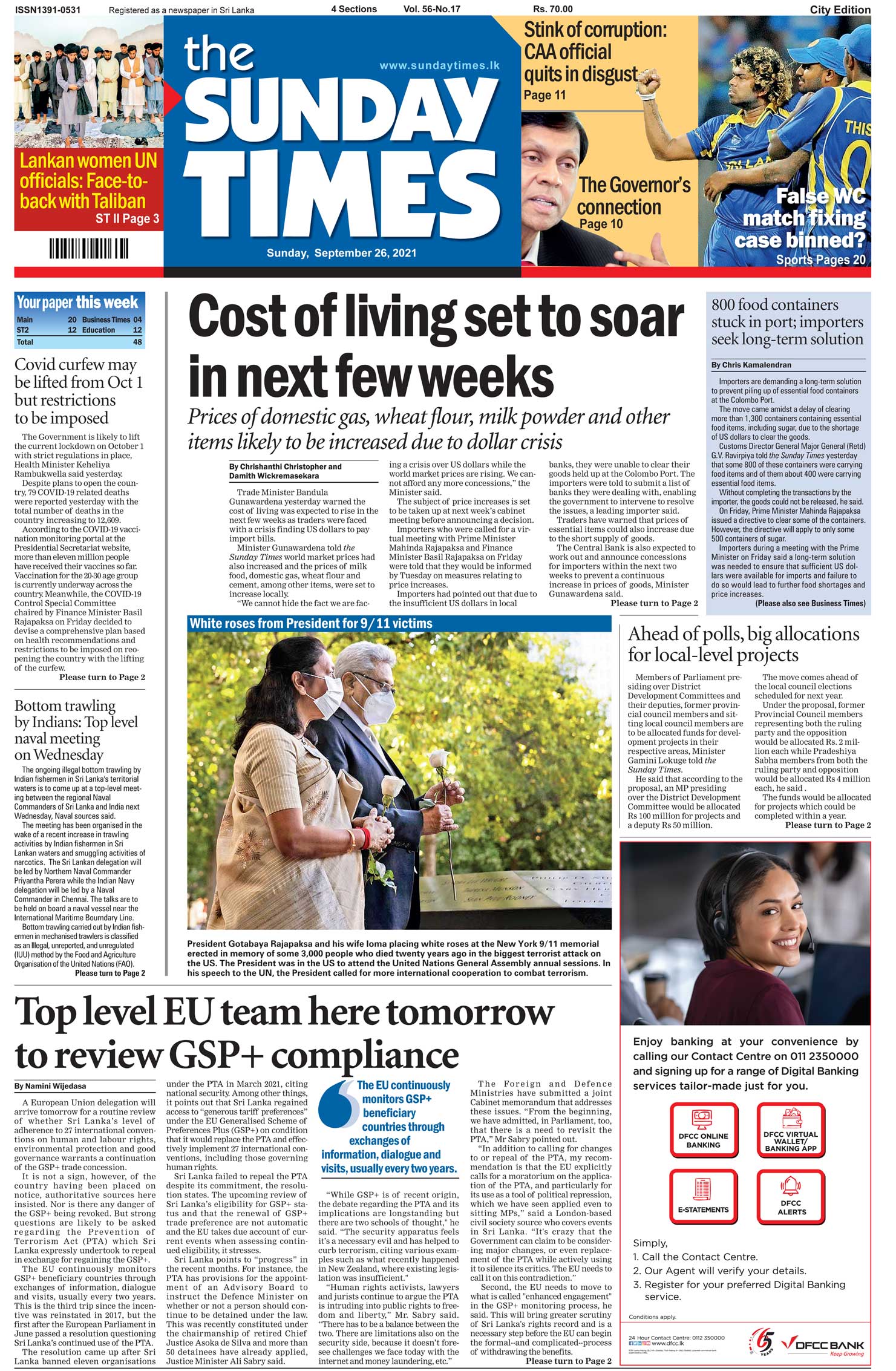**Detailed Caption:**

This image showcases a modern-day newspaper titled "The Sunday Times." The front page features a variety of headlines and articles accompanied by media images. The prominent headline reads, "Stink of Corruption: CAA Official Quits," directing readers to page 11 for further discussion. Adjacent articles include "The Governor's Connection," which can be found on page 19 or possibly page 12, and "False WC Match-Fixing Case Found?" with a question mark, highlighting an investigation involving players in blue uniforms accented with yellow.

On the side, there is an article focusing on a discussion involving Lankan women and UN officials, marked by a distinct bar separating it from other stories. Below the main title of the newspaper, a major headline warns, "Cost of Living Set to Soar in the Next Few Weeks," followed by a detailed subheading: "Prices of Domestic Gas, Wheat, Flour, Milk Powder, and Other Items Likely to Increase Due to Dollar Crisis." 

A central media image captures two individuals wearing masks at a 9-11 victims' rally, bringing an emotional touch to the page. At the bottom, another article announces, "Top Level EU Team Here Tomorrow to Review GSP Plus Compliance." Lastly, a media image of a smiling woman with headphones adds a lighter note to the diverse array of news presented.